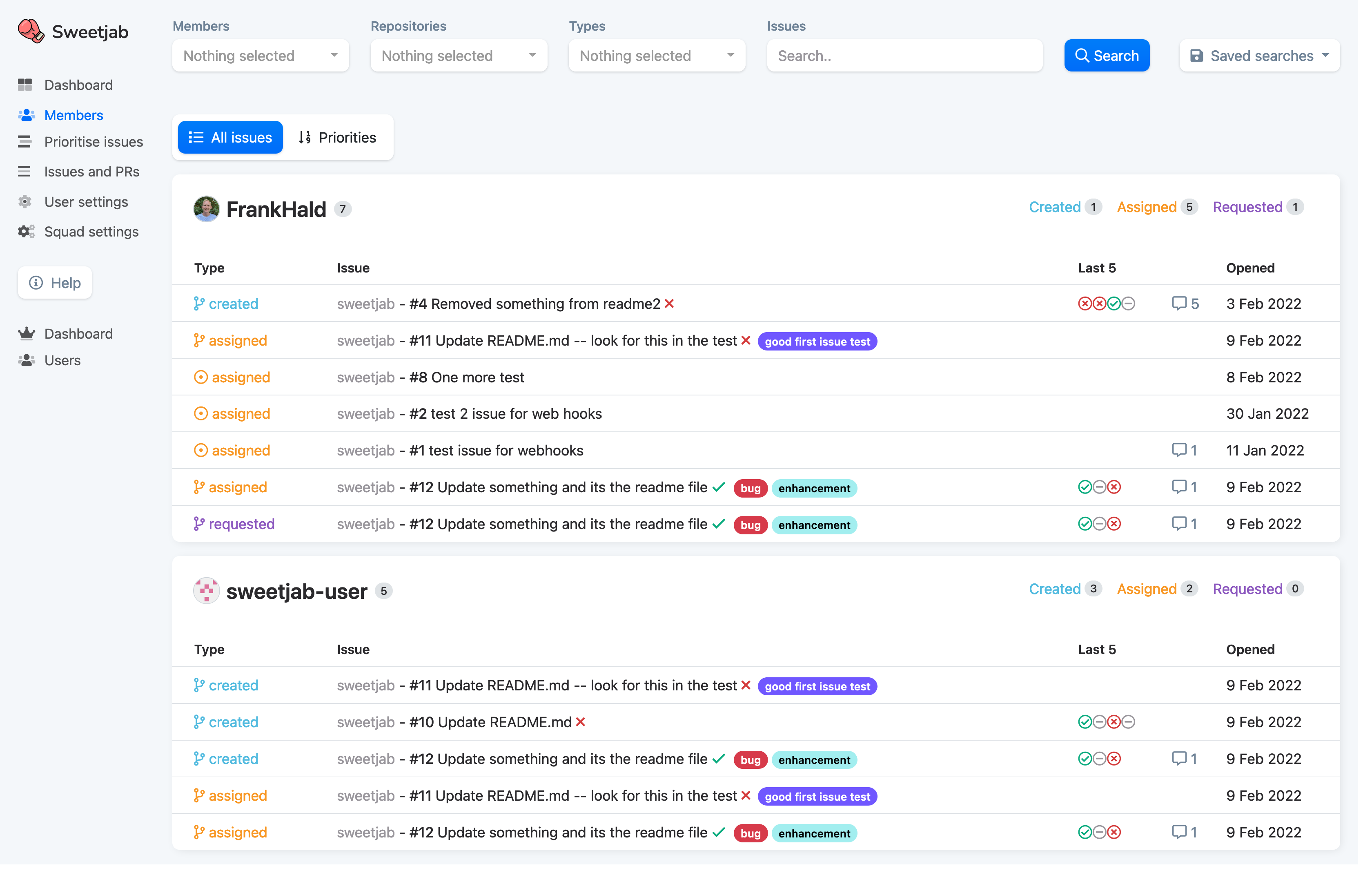This webpage screenshot, prominently labeled "Sweet Jab" in the upper left-hand corner accompanied by a relevant icon, centers around a comprehensive interface for managing projects and issues. At the top section, various drop-down menus are displayed: under the "Members" menu, no selection is made; similarly, the "Repositories" menu also shows "Nothing selected." To the right of these, another drop-down for "Types" is present but remains unselected. Adjacent to these menus is a search bar displaying placeholder text "search..." indicating where users can input queries. Next to this search field, a blue search button features a magnifying glass icon, signaling its functionality. Moreover, the "Saved searches" option, marked with a floppy disk icon, allows users to manage their saved queries.

The left sidebar lists an extensive navigation menu: "Dashboard," "Members," "Prioritize Issues," "Issues and PRs," "User Settings," "Squad Settings," followed by "Help," another "Dashboard" entry, and "Users." 

At the top right corner, it displays the user "Frank Hald," highlighted with a notification badge "7" next to his name, indicating outstanding notifications or tasks. Below this, labeled as "Sweet Jab - User," another user profile is visible, summarizing that individual’s details and project involvement.